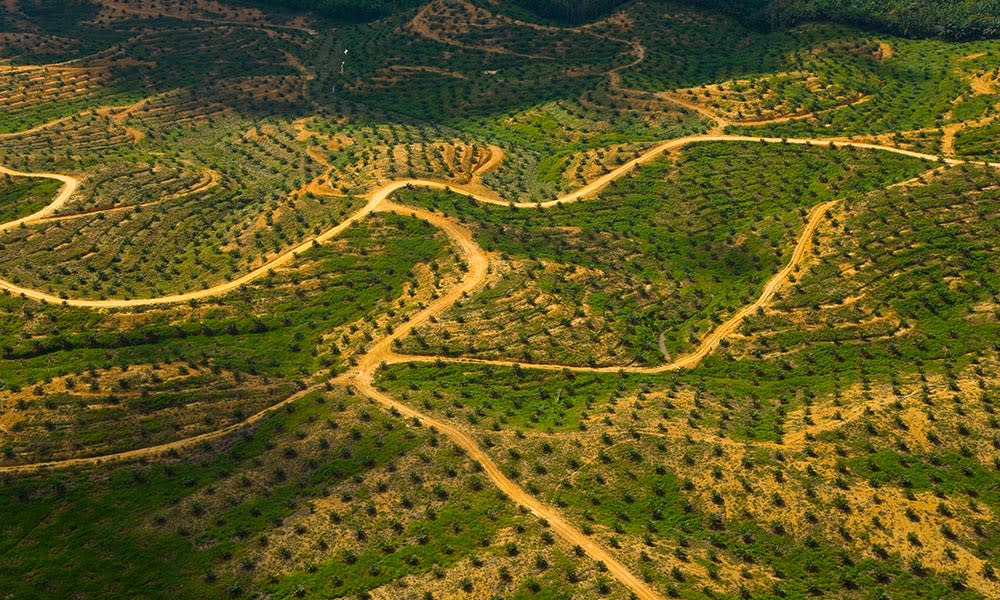The image is an aerial, sweeping shot of a hilly, grassy landscape interspersed with winding dirt paths. The rolling terrain is primarily green with patches of brown dirt, marked by numerous light brownish-orange dirt roads that cut through the scenery in a squiggling fashion. The photograph, taken in landscape mode with parts of it in shade, features orderly lines of dark green trees or bushes, spaced apart with remarkable symmetry, suggesting they might be cultivated. The landscape is devoid of any buildings or signs of civilization, emphasizing the natural and planned arrangement of the trees on the fields.